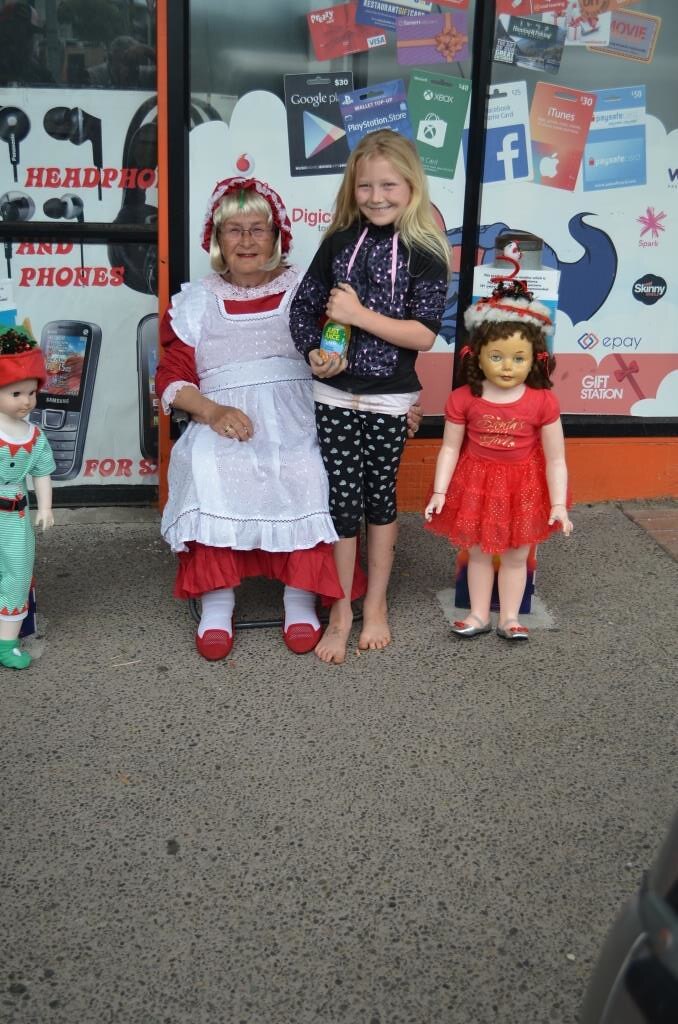In front of a storefront on the sidewalk, there is a detailed and vibrant scene featuring several objects and people. At the center of the image, an elderly woman is seated, wearing a costume consisting of a blonde wig, a red bonnet, a red dress with a white apron, white stockings, and red shoes. Standing beside her is a young girl with blonde hair, dressed in a black and white spotted outfit, and she is barefoot.

Flanking these two humans are two dolls in standing positions. The doll on the left is dressed in green clothing, resembling an elf costume with a blue and red outfit and a red hat. The doll on the right, placed directly next to the humans, has long hair in ponytails and is dressed in a white and red hat, a red dress, and white shoes.

Behind this central scene, various objects can be seen. There is a box of headphones and a collection of gift cards positioned in the back, displaying brands such as Google, PlayStation, Xbox, Facebook, and iTunes. The overall color palette of the photograph includes shades of light green, red, light red, tan, black, white, blue, yellow, purple, and orange. This vivid and eclectic arrangement seems to capture a moment outside a store, rich in detail and character.